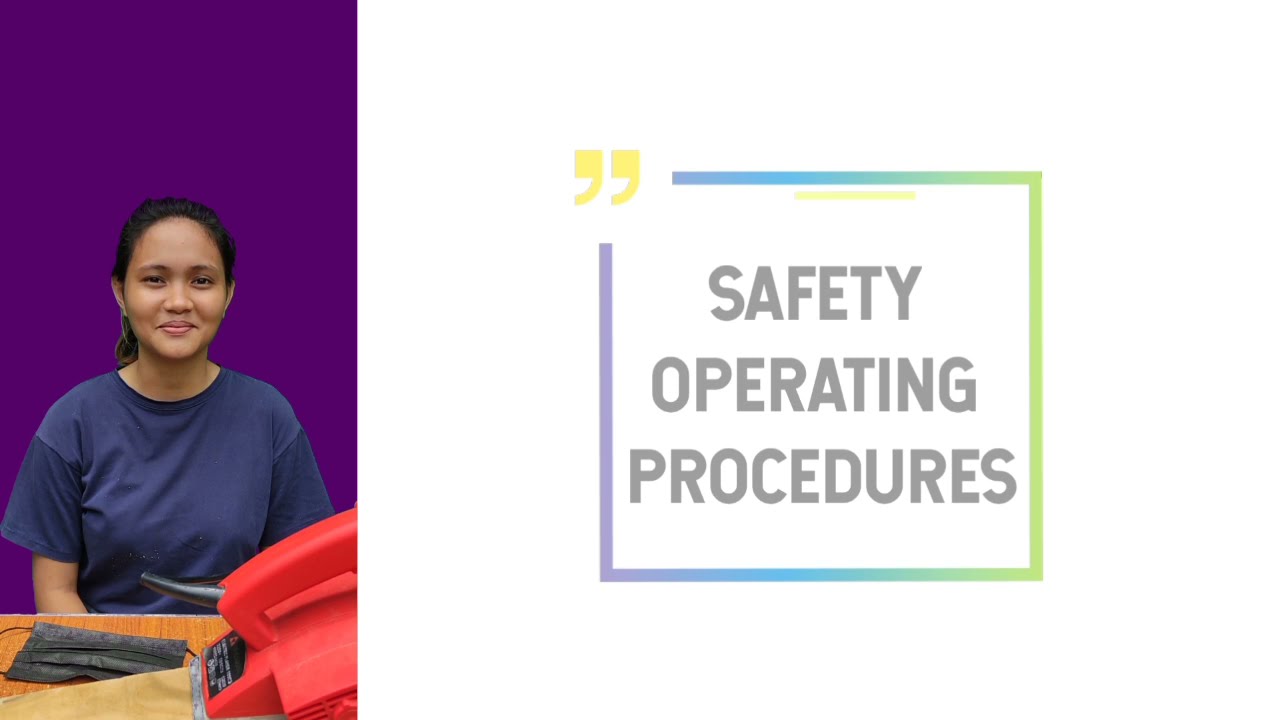The image depicts a woman seated at a rich wooden table. She is wearing a navy cotton t-shirt, short sleeve, and crew neck. She has caramel-colored skin, dark brown hair pulled back, dark eyes, notable cheekbones, a fleshy nose, and full lips. She is smiling slightly. In front of her on the table lies a black face mask with elastic ear loops, positioned on the rich, brown wooden surface. There's also a red power tool that resembles a sander, with a black cord protruding from its red handle, beside a beige piece of paper that looks like sandpaper. The background behind her is a purple color. To the right of the image, there's a sign with gray text reading "Safety Operating Procedures," bordered by a narrow, rainbow-colored frame. Yellow quotation marks are present at the top left corner of the sign, emphasizing the safety message.